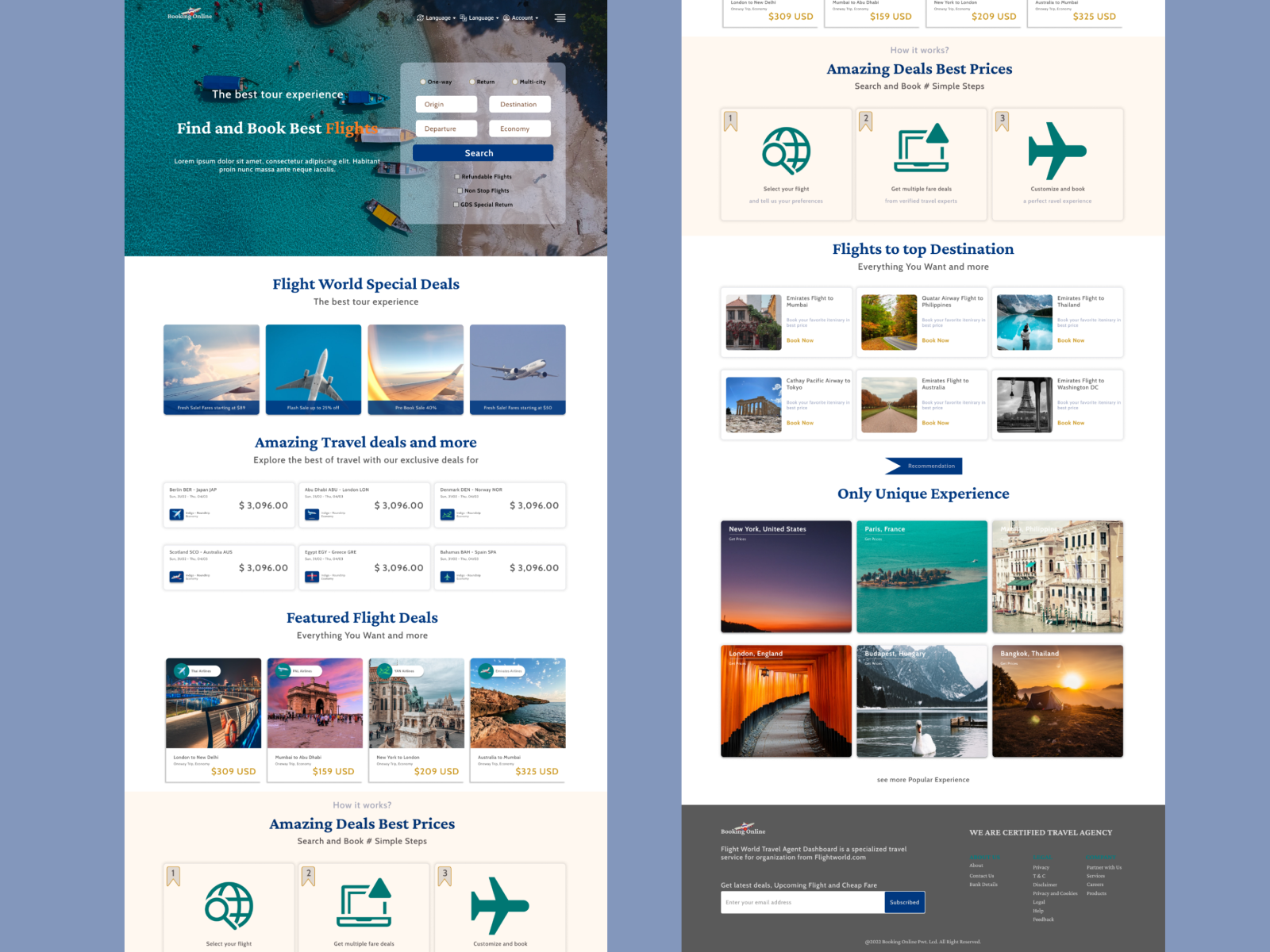The image features a meticulously designed rectangular background in periwinkle blue, upon which two distinct smartphone screenshots have been placed. The screenshots, which seem to be spaced deliberately to create a visually appealing layout, belong to what appears to be a travel company's website.

The left screenshot showcases the homepage of this travel platform. At the top, there's a sleek interface indicating options to find and book flights under the banner "The Best Tour Experiences, Find and Book Best Flights." A captivating aerial photo depicts several small boats in a striking blue sea. Below this, users can interact with various input fields labeled "Place of Origin," "Destination," "Departure," and "Class" (e.g., Economy), all designed for a seamless flight search experience.

Continuing down, the page is segmented into sections that enhance usability and visual interest. The first section hosts the mesmerizing photo followed by four smaller images of exotic locations. Then, it highlights “Amazing Travel Deals” with an assortment of flight deals, each represented by visually appealing photos and price points starting at $3,096. The next section, titled "Featured Flight Deals," presents four more snapshots of popular destinations, emphasizing the best prices and offers available. At the bottom of this screenshot, there's a footer replete with additional links and a search bar.

The right screenshot appears to continue the user experience from the left page, showcasing further travel offers. It features additional alluring imagery of top destinations, again split into neatly organized sections, each with six enticing photos. The section at the bottom highlights "Only Unique Experiences," complemented by a series of larger images, inviting users to explore bespoke travel packages. The footer echoes that of the left screenshot, complete with a search bar and the company's logo, providing a cohesive end to the visual journey.

Overall, the image effectively portrays a user-friendly, aesthetically pleasing snapshot of a comprehensive travel booking website designed to entice and inform prospective travelers.